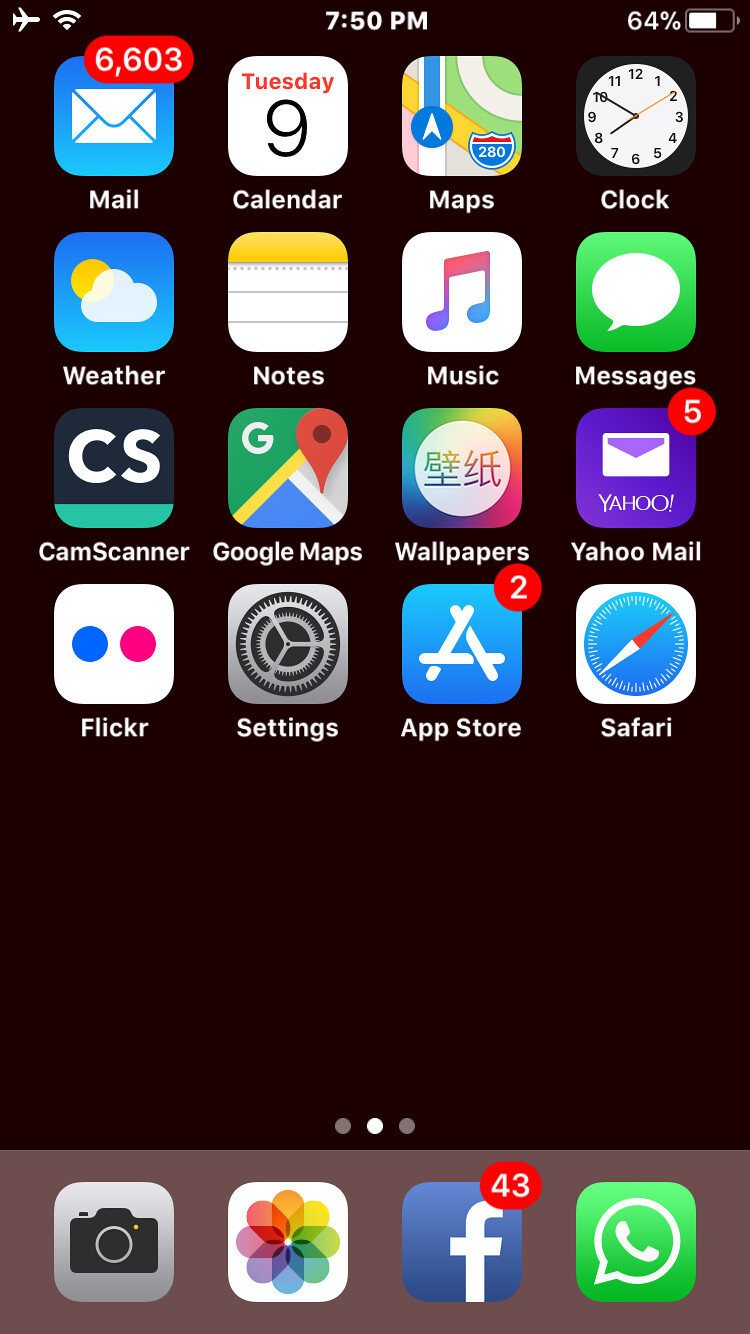This is a screenshot of an iPhone home screen displaying the following details:

- At the top of the screen, there are various status icons: the Airplane Mode icon, the Wi-Fi icon, the current time (7:50 PM), and the battery indicator showing 64% alongside the battery icon.
- The Mail app icon is blue with a white envelope and has a red notification badge displaying 6,603 unread emails.
- The Calendar app icon shows the date "Tuesday 9."
- The Maps app icon features a map design, while the Clock app icon has a black clock with a white center.
- The Weather app icon depicts a cloud and sun.
- The Notes app icon looks like a notepad with a yellow top.
- The Music app icon displays a musical note.
- The Messages app icon is also present.
- Next is the Scanner app with "CS" labeled.
- The Google Maps app icon features a "G" and a map pin.
- An app with a Wallpapers icon contains Chinese characters.
- The Yahoo Mail app icon is purple with a white envelope and has a red notification badge showing 5 unread emails.
- The Flickr app icon is a white square with two circles (one blue, one pink).
- The Settings app icon, the App Store icon with a red notification badge showing 2 updates, and the Safari app icon, which shows a compass, are also displayed.
- Additional icons include:
  - The Camera app
  - The Photos app
  - The Facebook app, which has a blue square with a white "F" and a red notification badge showing 43 notifications.
  - The WhatsApp app icon.